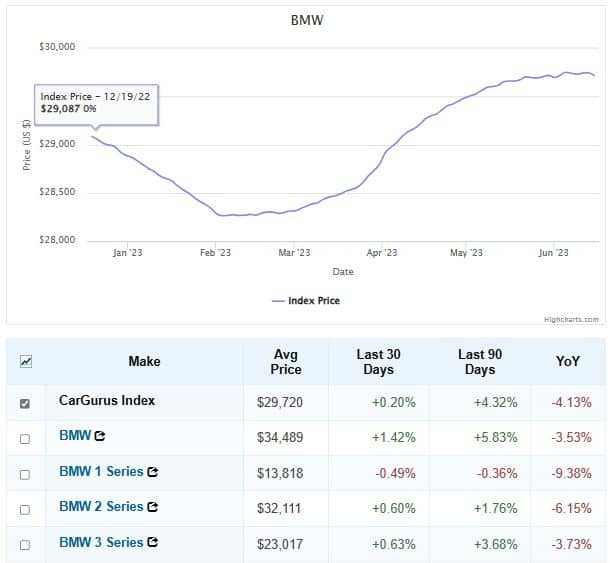A detailed caption for the described image could be:

"This image features a line chart with a plain white background, appearing as a screenshot. Centered at the top in dark gray capital letters is the title 'BMW.' Directly underneath this title is the top boundary line of the chart, marked at $30,000, while the bottom boundary is at $28,000. The starting index price of the chart is notably high, beginning at 29,087%. The chart spans vertically between these monetary values, representing the price ranges.

The line chart is part of the 'CarGurus Index,' as stated by the large, bold title also centered at the top, just below the BMW heading. This area is shaded with a light blue rectangle for visual emphasis. The chart comprises multiple entries, each represented by a separate line and label positioned to the left. The entries include, in order: 'BMW,' followed by specific series such as 'BMW 1 Series,' 'BMW 2 Series,' and 'BMW 3 Series.' Towards the lower section of the chart, various lines denoting different data points contribute to a detailed and comprehensive depiction of the car index values."